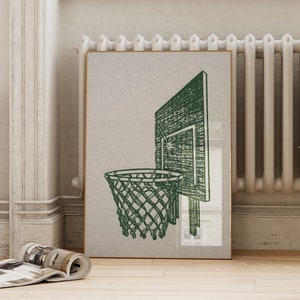The photograph captures a framed piece of art propped against a traditionally styled white radiator, which is mounted on a similarly white wall. The artwork is encased in a light blonde wood frame and covered by glass. It features a black-and-white drawing of a basketball and a hoop with a net, depicted from a side angle. Notably, the backboard of the hoop includes an inner square, in the corner of which a sun-like design is illustrated. The flooring beneath the artwork is made of light blonde wood, matching the frame, and prominently features a folded magazine. The magazine, partially tucked under its own fold, is positioned at the base of a square-post-style wooden column.